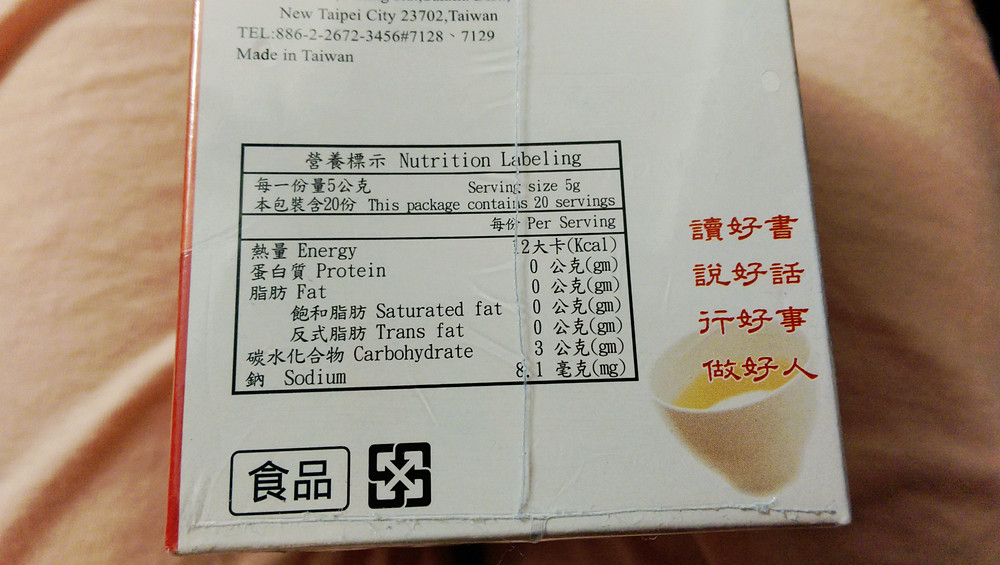The image features the back of a coffee product box positioned on a slightly wrinkled peach-colored sheet. The box casts a shadow to its right. In the upper right-hand corner of the image, a small portion of a black object is visible. The box itself is predominantly white with a thin red border running along its left side. A faint thread-like line runs down the middle of the box. 

In the lower right corner of the box, there is an image of a white cup containing a yellowish liquid, possibly tea, accompanied by red Chinese characters. Additionally, there is a black section with nutritional information, stating that the serving size is 5g, the package contains 20 servings, and each serving provides 2 kilocalories. The nutritional details also list 0g of protein, fat, saturated fat, trans fat, and carbohydrates, with a sodium content of 8.1mg.